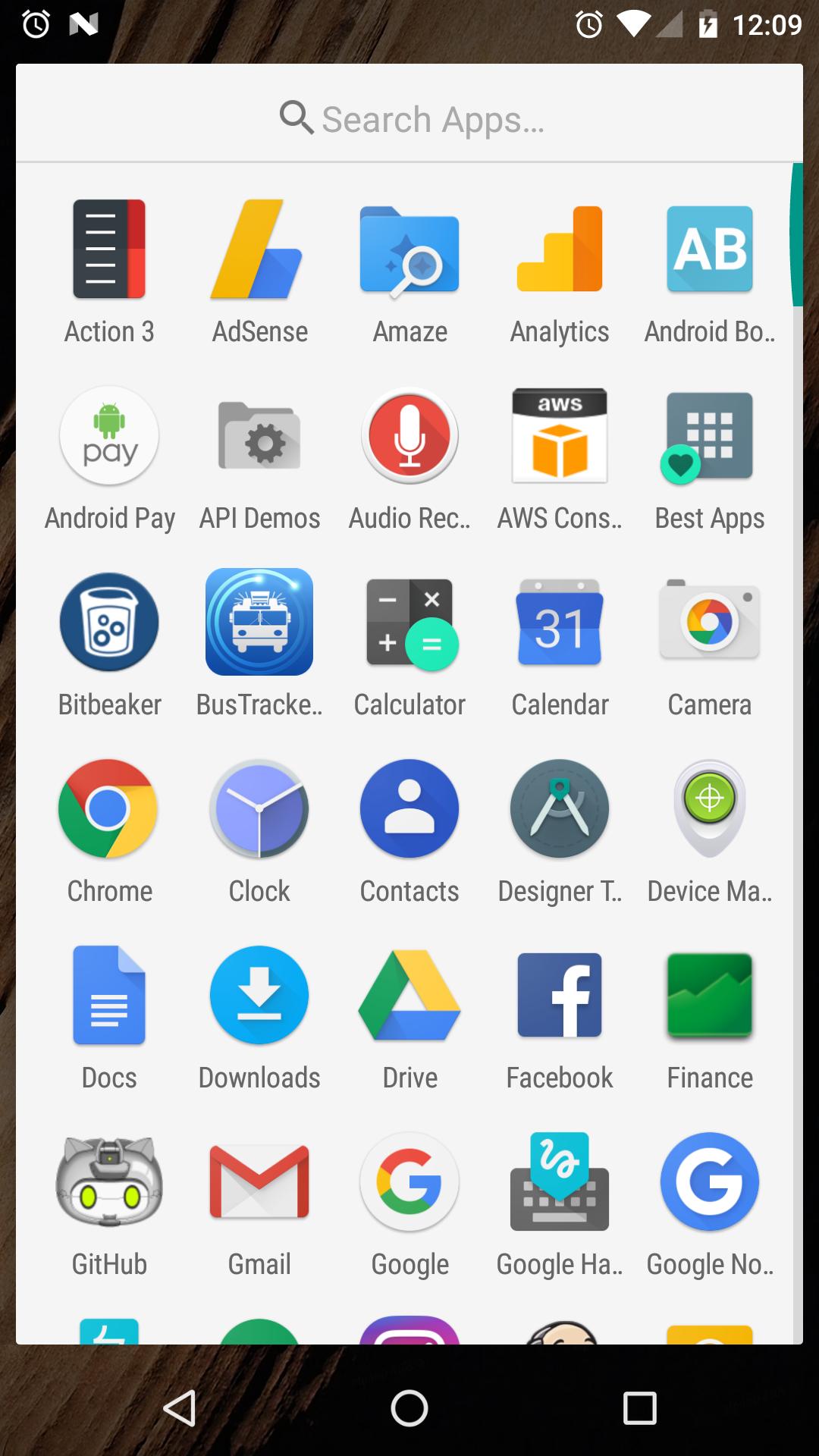The image depicts the home screen of an Android smartphone filled with a variety of colorful app icons. At the top of the screen, there is a search bar labeled "Search Apps." The apps are arranged in a grid pattern, starting with "Action 3," followed by "AdSense," "Amaze," "Analytics," "Android B," and so on. Notable apps include "Android Pay," "Gmail," "Finance," "Facebook," "Drive," and "Downloads," each represented by distinct and vibrant icons. The "Analytics" app is particularly striking with its gradient of yellow hues transitioning to a rusty orange color. The layout and design are typical of an Android device, which may appear unfamiliar to those accustomed to other operating systems.